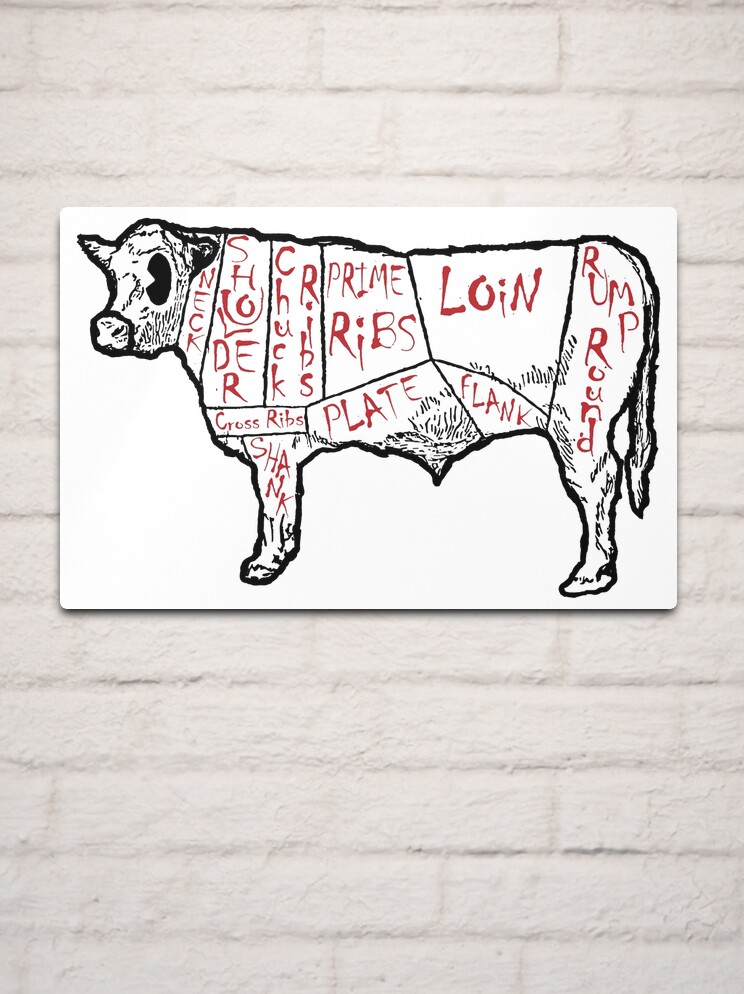The image depicts a detailed butcher's chart of cuts of meat on a steer, set against a very light gray brick wall that's been painted. The horizontal rectangular poster features a white background with a line drawing of a cow in profile, marked by black lines that outline the various cuts of meat. Each cut is labeled in a distinctive handwritten red font, reminiscent of blood, spanning from the neck to the rump. The cow illustration includes labels such as loin, rump, round, flank, plate, prime ribs, chuck ribs, short ribs, cross ribs, shank, and neck. The steer drawing showcases some texture, adding depth to the image. The chart appears to be either paper or metal and is affixed to the wall, which displays the characteristic textures and patterns of bricks.